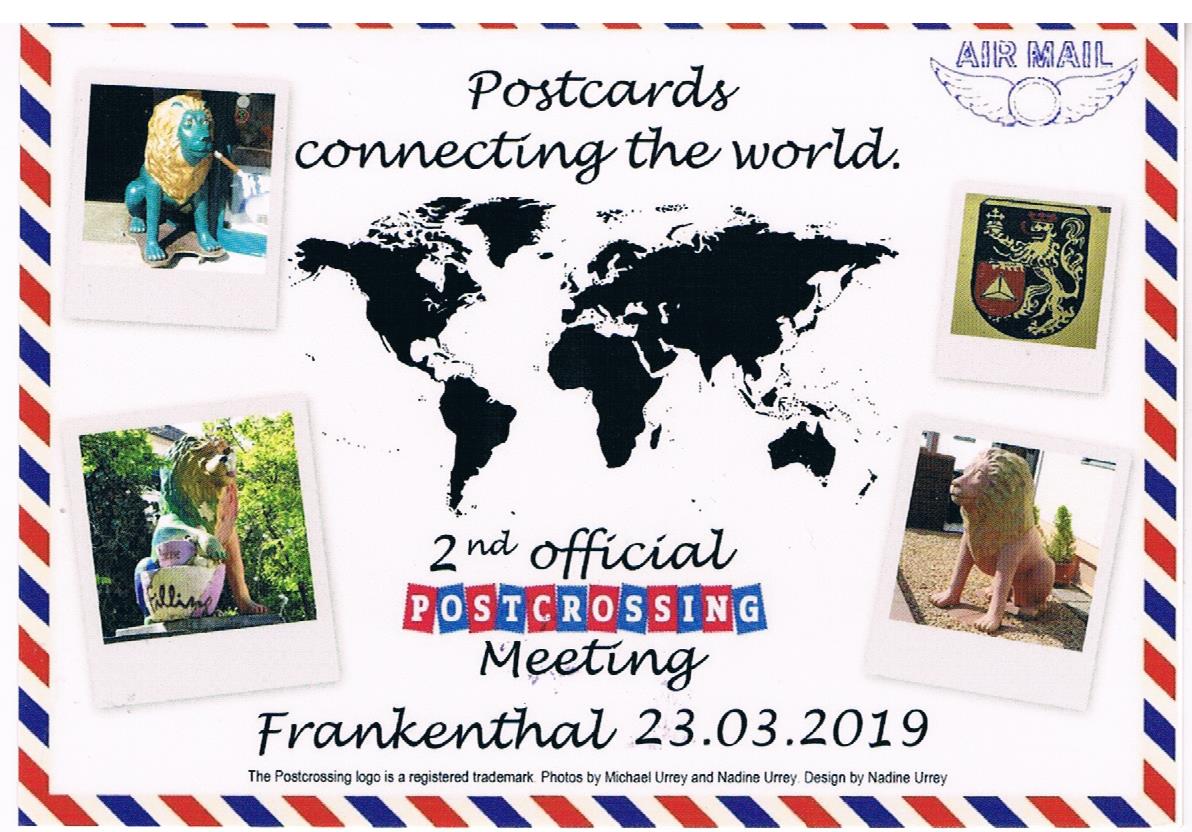The image showcases a detailed postcard with a diagonal red, white, and blue striped border. The background is white, and prominently featured in the upper right corner is a blue stamp marked "Air Mail" with wing symbols. At the top center, the heading "Postcards Connecting the World" is displayed in black. Below this title, in the center, is a black silhouette of the world map. Flanking the map are four Polaroid-style photos depicting various lion statues and emblems, with two photos on the upper left and right, and two on the lower left and right. Under the map, the caption reads "Second Official Post Crossing Meeting" in black. Following this, in alternating red and blue squares with white lettering, is the "Post Crossing" logo, a registered trademark. Below the logo, additional text states "Meeting" and "Frankenthal 23.03.2019." The design credits reveal that the postcard was designed by Nadine Urey, with photos taken by Michael Urey and Nadine Urey.